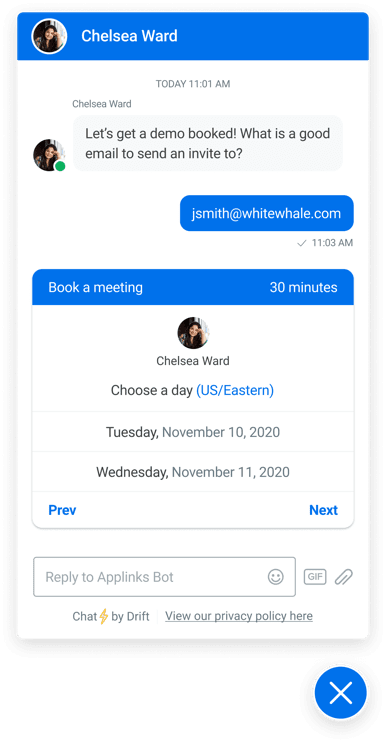A detailed descriptive caption for the image could be:

"In this screenshot of a social media account chat, Chelsea Ward is attempting to book a meeting. At the top, 'Chelsea Ward' is prominently displayed. Below, there's an image of a woman with dark hair likely Chelsea herself. The accompanying profile picture denotes the current time as 11:01 AM, with Chelsea Ward stating, 'Let's get a demo booked. What is a good email to send an invite to?' Following this, an email address 'jsmith@whitewhale.com' is visible, timestamped at 11:03 AM, with an option to 'Book a meeting for 30 minutes.' The profile picture of Chelsea Ward appears again, and underneath, a prompt to choose a day in U.S. Eastern time zone is available, listing dates Tuesday, November 10th, 2020, and Wednesday, November 11th, 2020, with navigation buttons 'Previous' and 'Next.' Towards the bottom, there is an input box to 'Reply to Applinks bot,' featuring a smiley face emoji, a GIF option, and a paperclip symbol for attachments. Finally, the bottom section includes chat options with a lightning symbol by Drift, a link to view the privacy policy, and a blue circle with a white 'X' at the very bottom."